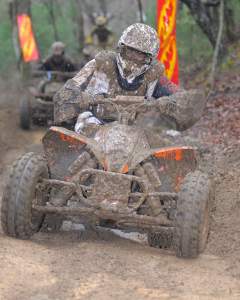This daytime outdoor scene depicts a mud-splattered race involving off-road vehicles on a narrow, muddy trail. In the foreground, a rider on a predominantly orange and white ATV, completely covered in light brown mud, wears a white helmet and a mask. The trail is flanked by red, orange, and yellow flags, with blurred green foliage and a prominent tree trunk visible on the right side. Flying mud and blurred greenery add to the dynamic action as two additional ATV riders, equally mud-covered, trail behind the main rider. Rectangular red and yellow signs with indistinct logos line the sides of the path, enhancing the sense of a competitive race through this rugged terrain.